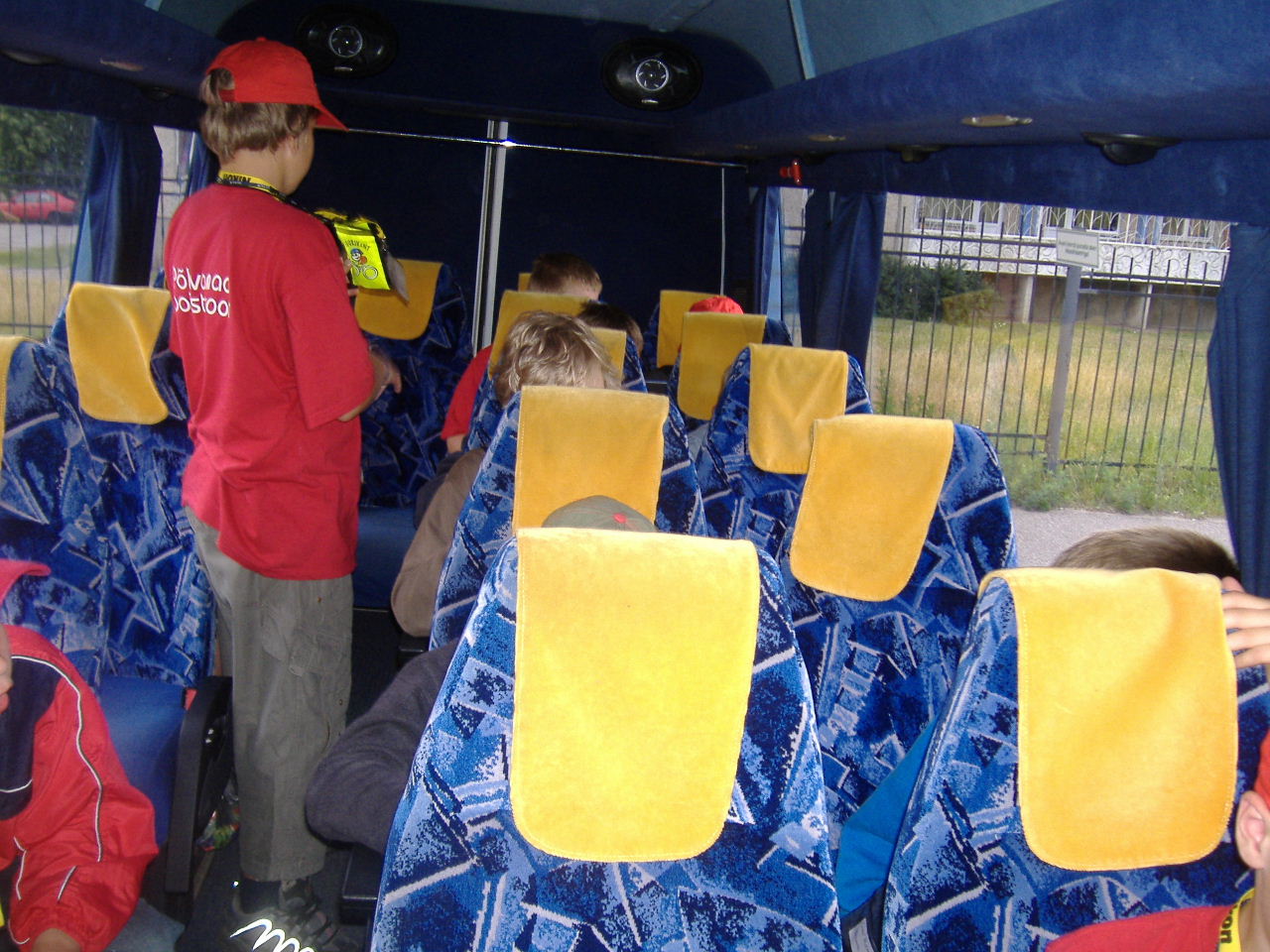The photograph captures the inside of a bus adorned with blue and white patterned seats, each with a golden-yellow cloth draped over the top. The viewer's perspective is from the front, looking towards the back of the bus, which features a dark blue panel. Prominent in the center is a young boy facing away from the camera, wearing a red short-sleeve t-shirt with white writing, gray pants, black sneakers with black shoelaces, and a red baseball cap over his short dirty blonde hair. He appears to be holding a clipboard and possibly talking to one of the kids seated nearby. Surrounding him, you can see the tops of other children’s heads, some donning baseball caps in red and gray. Towards the lower right corner, a child in a red jacket with a white stripe on the sleeve is partially visible. Through the bus's clear right-side window, a gray wrought iron fence and a white building can be seen against a green lawn, adding a touch of the outside world to the scene inside the bus.